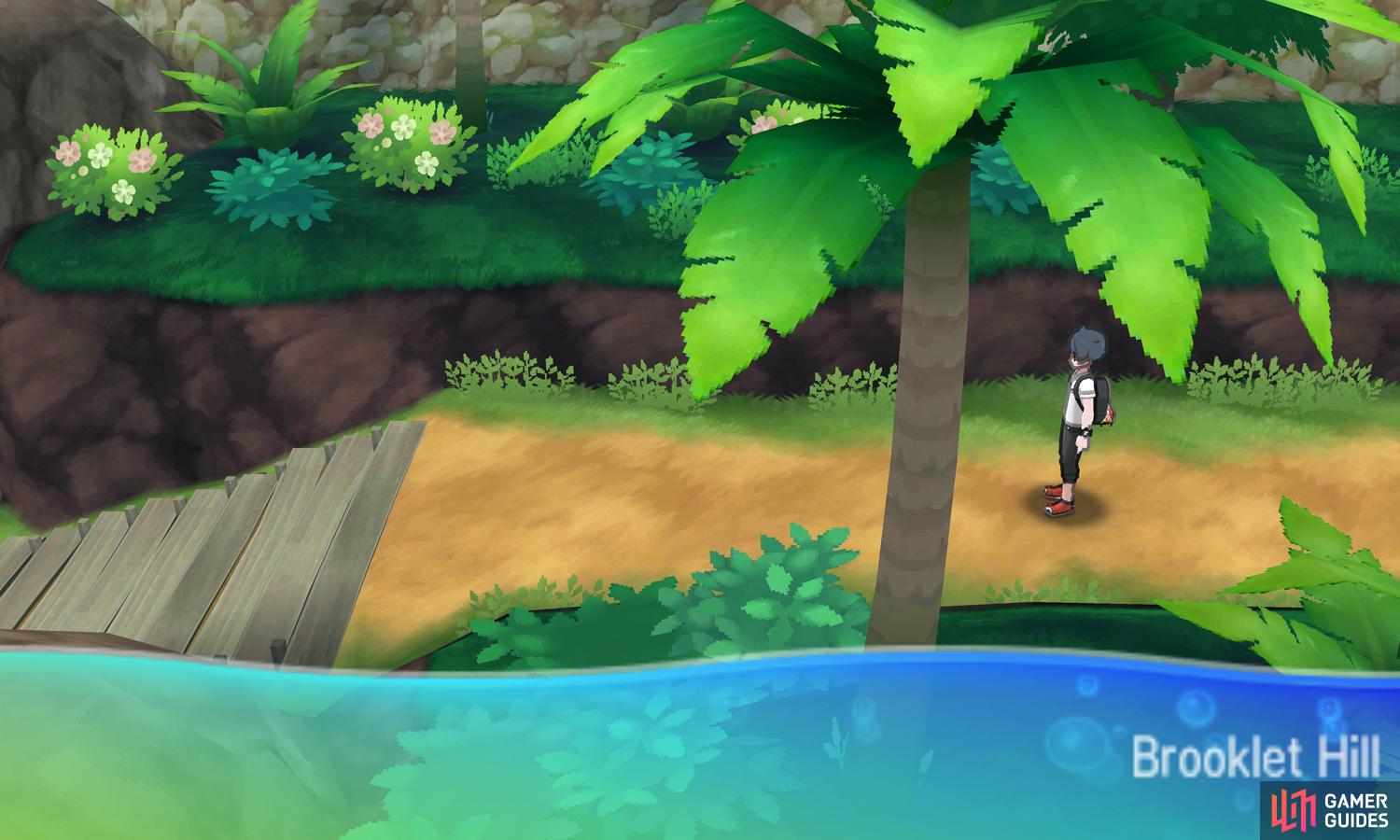This image is a screen capture from a Pokémon video game, depicting a detailed and vibrant in-game environment. Centered around a path, the scene features a character on the right side who has blue-gray hair, wears a backpack, greenish khaki shorts, red shoes, a white shirt, and a watch. This character stands facing partly away from the viewer, either walking or idling on the path. In the foreground, a pixelated palm tree extends from the bottom to the upper right corner of the image. The left side of the path ends at a brown wooden bridge or walkway that appears to go over a cavern. Surrounding the path, there are patches of grass and high shrubs adorned with pink and white flowers. In the background, additional greenery and ledges with bushes are visible. Overlay text in white letters at the bottom right reads "Brooklet Hill," and below it, "Gamer Guides" is prominently displayed, confirming the illustrative game setting.